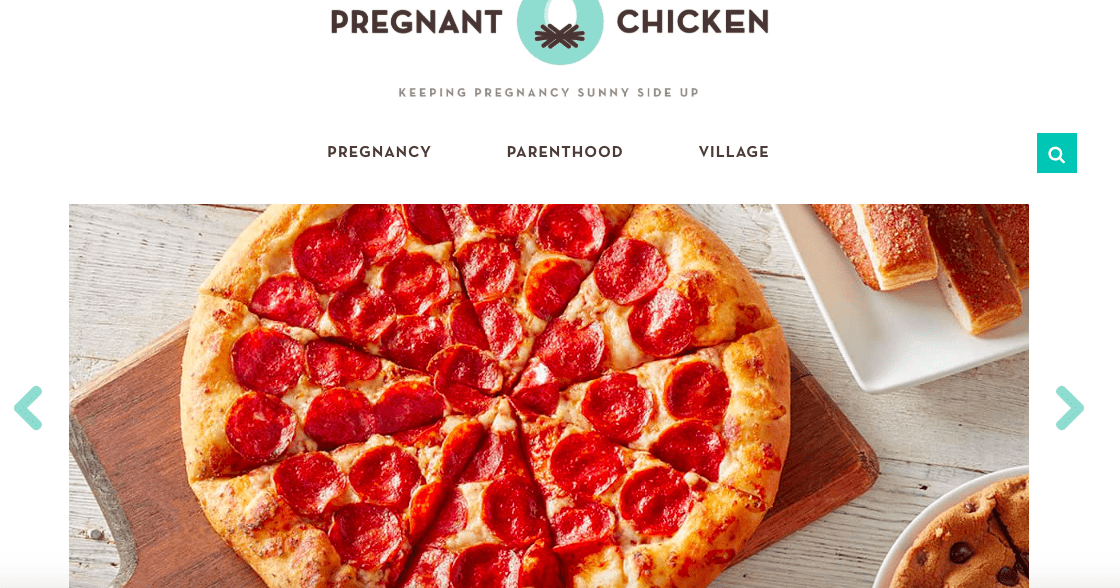On a white background, the top part of the image features the text "Pregnant Chicken" in dark brown, with capital letters. Between the words "Pregnant" and "Chicken," there is a partially obscured turquoise "O" with a white center. The bottom of the "O" resembles small brown logs, reminiscent of firewood. Directly below, in small brown letters, the caption reads "Keeping Pregnancy sunny side up," followed by "Pregnancy, Parenthood, and Village" in larger brown text.

To the right of this text, there is a small green box containing a white search icon. The main image displays a large pizza on a brown cutting board, placed on what appears to be a beige wooden surface, painted to look like a picnic table. The pizza has a thick, doughy crust, covered generously with cheese and pepperoni. Next to the pizza, a white porcelain plate holds what seem to be breadsticks sprinkled with sesame seeds. Another white plate showcases a large chocolate chip cookie. Additionally, a small green arrow pointing to the right is located to the right of the image, above the white bottom section of the background.